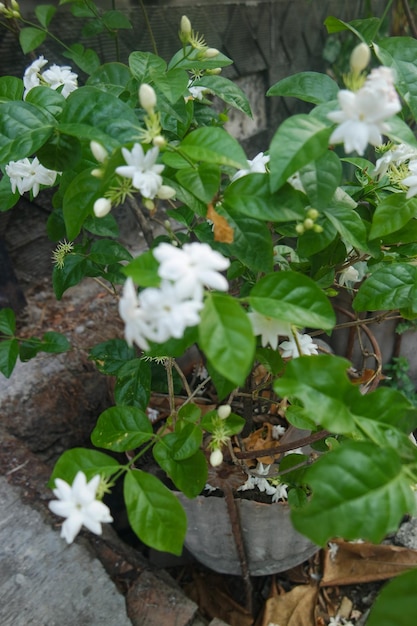This rectangular photograph captures a vibrant green plant thriving in a gray, stone pot set outdoors. The image, taken from an elevated angle, showcases the plant's healthy green leaves and a profusion of small white flowers with tiny yellow centers, facing in all directions. Some flowers are in full bloom, while others are wilting or still budding. Fallen dead flowers are also visible around the plant. The container rests in a rocky and dirt-filled landscape, with some cement in the foreground, suggesting a designated planting area. A tree trunk is faintly discernible in the background, although much of the surrounding environment appears out of focus due to the tight zoom on the plant itself. The overall scene highlights a mixture of life stages within the plant, from fresh buds to mature blooms and foliage.